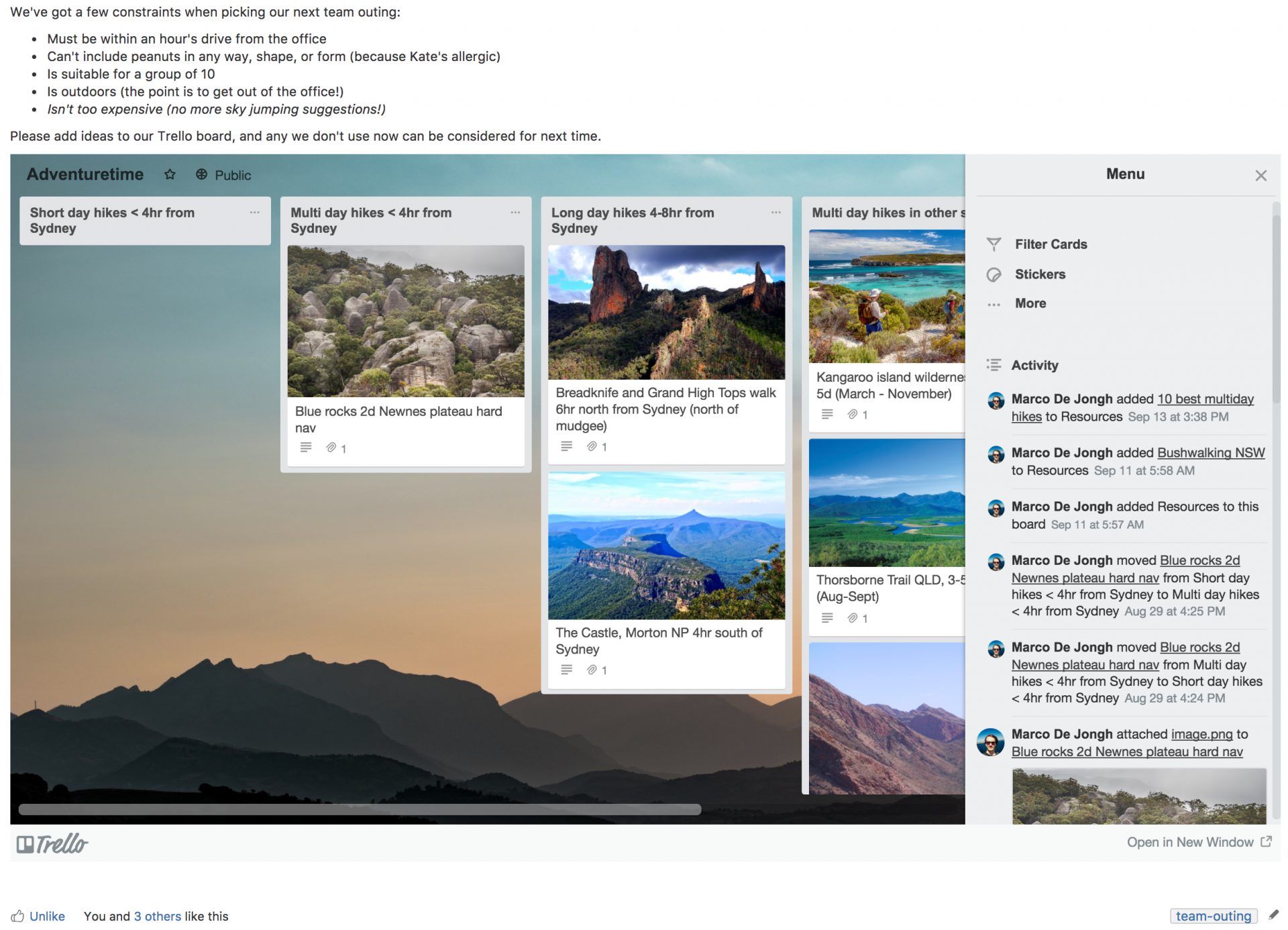The image contains a densely packed layout with several sections and elements, which can be broken down and described in detail as follows:

At the top of the image, there is a small, indistinguishable line of writing. Below this, a sentence is followed by five bullet points, accompanied by another line of writing beneath them. 

The main focal point of the image includes a visual scene depicting a sky and mountains in the background, with "Adventure Time" written prominently at the top. Adjacent to this, there is a black-outlined star, a circle featuring some black coloration, and the word "Public" written inside the circle.

On the left-hand side:
1. A white rectangle containing text that is too small to read.
2. Below this rectangle, there is a longer grey-bordered rectangle. At the top of this grey-bordered rectangle, there is some writing that is not legible. Inside this rectangle, there is an image showing what appears to be large rocks, with another white rectangle beneath it containing small, illegible text. 
3. Another grey-bordered rectangle below, containing an image that depicts rock formations or hills against the sky, with a white rectangle underneath featuring small, unreadable text.
4. A third image beneath that shows the sky and blue hills, accompanied by a white rectangle with unreadable text.

There are additional sections with fragmented images partially cut off. These sections include a picture, a portion of a white rectangle with writing, and three other similar image segments without any legible text beneath the bottom picture.

Towards the bottom right:
1. A grey rectangle marked "Menu" at the top, with a close (X) button on the right.
2. Various icons and options inside the rectangle, including a funnel icon labeled "Filter Cards", an icon labeled "Sticker", three dots in a row labeled "More", and some lines labeled "Activities".
3. Six small unidentifiable circular images, with the last and largest one possibly containing a person's face. Each of these circular images has adjacent writing that is too small to read.
4. Part of a picture is visible at the bottom, followed by more blue-colored writing that is also unreadable.